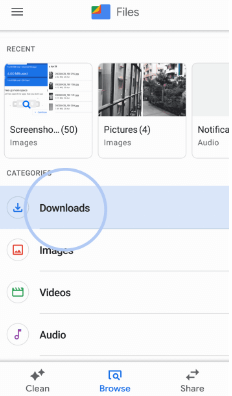Screenshot of a Tablet/Smartphone Interface:

At the top left of the interface, within a light gray rectangle, there is a dark gray icon depicting three horizontal lines, indicating the settings menu. Nearby, there's an icon labeled "Files" in either dark gray or light black text. This icon features a stylized green corner, creating an effect as though the paper or folder's corner is peeling away and bending to the right. Sequentially, the following icons are orange, red, and then dark blue.

Underneath this, there is a thin dark gray shadow and, written in black, the word "Recent" appears. Several thumbnails of screenshots are visible below. The first screenshot on the left shows an area of blue alongside white, and appears to be an interface displaying various screenshots and information. The title reads "Screen" followed by the truncated text "Screen Sho..." and includes "50" in parentheses. Below this text, in gray, it says "Images.”

The contents of the screenshot depict a side of a building with numerous windows, black bracers, white edges, a tan and white building in the background, dark green bushes, and a concrete path. Next to this, there is a section labeled "Pictures" in black with "4" in parentheses, and below it "Images" in gray.

Further down, there's a partially visible section labeled "Notifications," followed by "Audio." In the lower portion of the screen, there is a gray label "Categories." Highlighted among various rectangles is a blue-shaded one, signifying it’s currently selected. This rectangle features a gray circle with a dark blue arrow pointing to a fraction of an open square. Next to it, under a baby blue circle labeled "Downloads" in bold black text, there's another light gray bordered circle with an orange square depicting the silhouette of mountains. Bold black text next to it reads "Images."

Subsequently, another green icon illustrates a calendar or movie clapper, labeled "Videos." A purple music note icon is also visible with the text "Audio" next to it. On the lower left-hand edge of the device's bezel, there are two adjacent dark gray or black diamonds labeled "Clean" in dark gray. Adjacent to this, part of a magnifying glass icon in blue says "Browse," indicating the current selection.

On the right-hand side of the screen, two arrows, one pointing left and the other right, are colored in dark brown, gray, or black. Below these arrows is the word "Share" in dark gray.